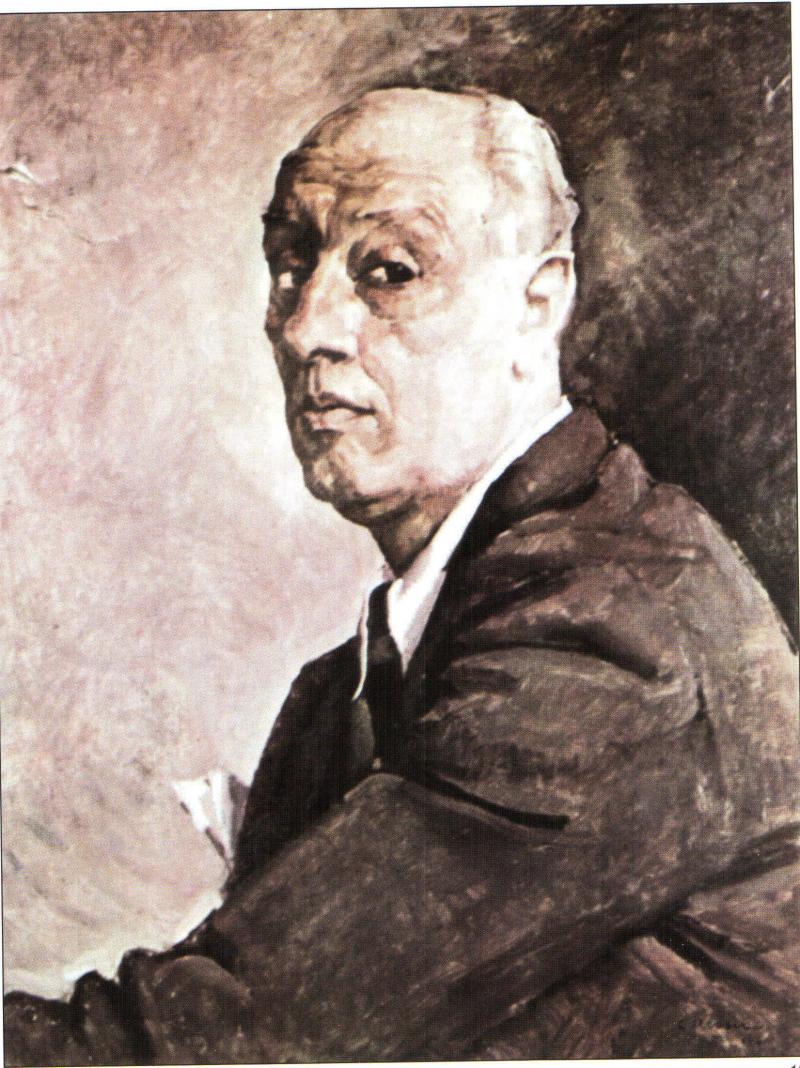This is a detailed painting titled "Self-Portrait" by Camille Ressu. The artwork portrays an elderly man, likely between 60 and 70 years old, with a distinctive look of skepticism on his face. His raised eyebrows, finely accentuated wrinkles, and dark shadows under his eyes contribute to a tired yet piercing expression. The man, a white gentleman with a receding hairline and gray hair on the sides, is depicted looking directly at the artist, suggesting he posed for this piece. He's dressed in a dark suit, white dress shirt, and a black tie, all rendered in various shades of black, white, and gray, with subtle sepia tones adding depth to the otherwise monochromatic palette. The background features reddish-brownish hues and a mix of black and light gray brushstrokes, creating a textured and dynamic backdrop. His neutral expression and the meticulous detail in his attire and facial features make this a compelling and introspective self-portrait.